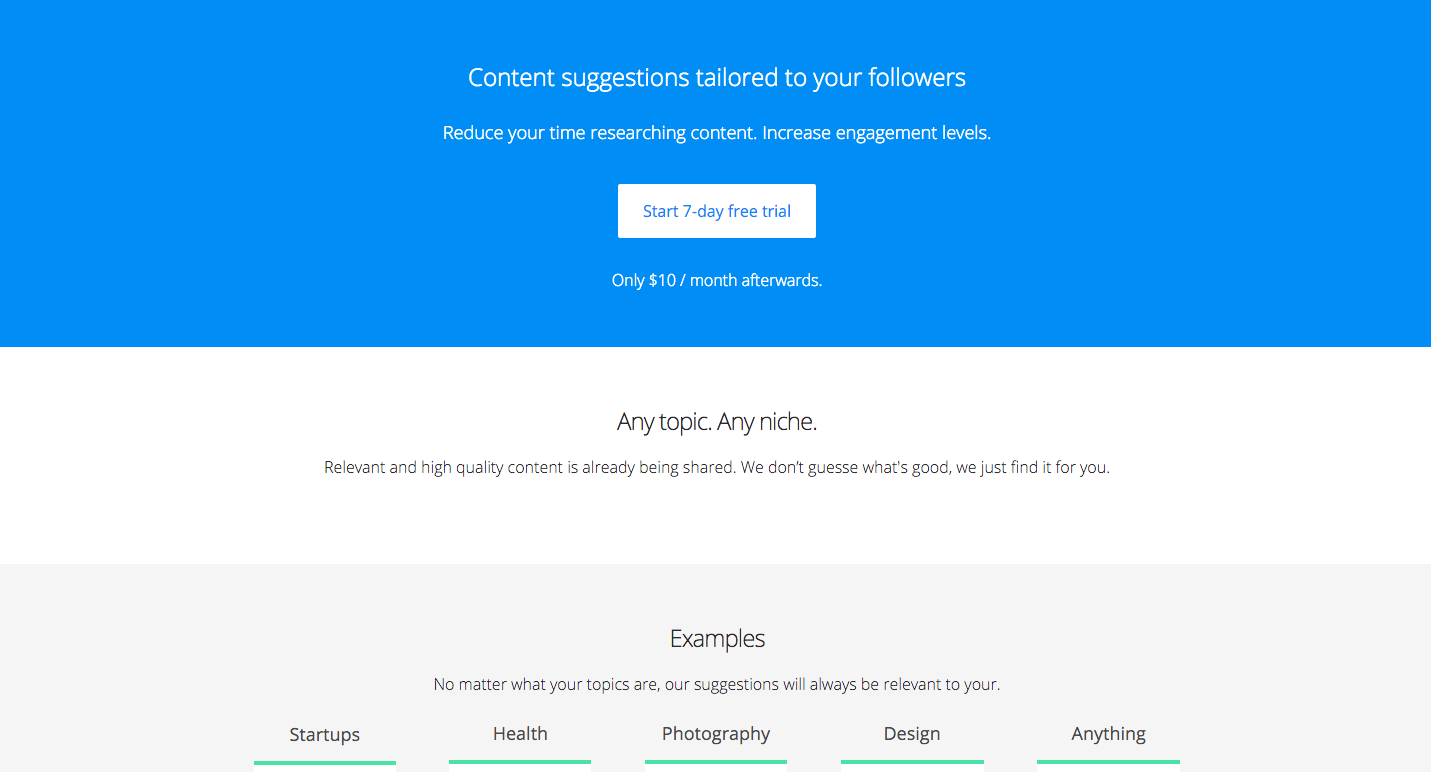A promotional graphic with a light blue background occupies the top portion of the image. Centered within it, white text reads: "Content suggestions tailored to your followers. Reduce your time researching content. Increase engagement levels." Below this text, a rectangular button prompts with: "Start 7-day free trial" and includes the cost details: "Only $10 a month afterwards."

Further down, a section with a white background features black text stating: "Any topic, any niche. Relevant and high-quality content that's already being shared. We don't guess what's good; we just find it for you." 

Underneath this, another rectangular box in light gray is centered and contains black text which reads: "Examples: No matter what your topics are, our suggestions will be relevant to you."

At the bottom section, several clickable options are listed—"Startups," "Health," "Photography," "Design," and "Anything"—each separated by thin teal-colored horizontal lines.